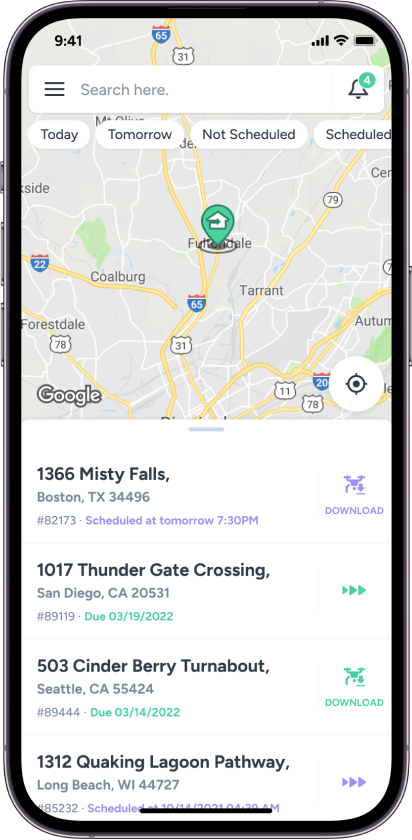"An intricately detailed map showcasing various geographical locations and numeric data. The image includes locations like Misty Falls, Austin, Texas with coordinates C1366, and Quaking Lagoon Pathway, Long Beach, WI, identified by the number 44727. It is evident that the destinations include commercial sites such as a 'hamburger banger' represented by a bell icon on map location four. There are three arrows pointing to directions labeled with numbers like 85232 and 503, indicating potential routes or areas of interest. The map also features a full signal indicator and a fully charged battery icon. Additionally, schedule times are mentioned, such as a pin scheduled for tomorrow at 7:30 PM in San Diego, California, with coordinates 20531, and another marker in Austin, Texas listed for 10:17:30 AM. The imagery is likely intended for a detailed logistical or navigational purpose, with various codes and identifiers like 'Colbert for a Zell turn' and 'Cinderbury turnabout' further enriching the content."